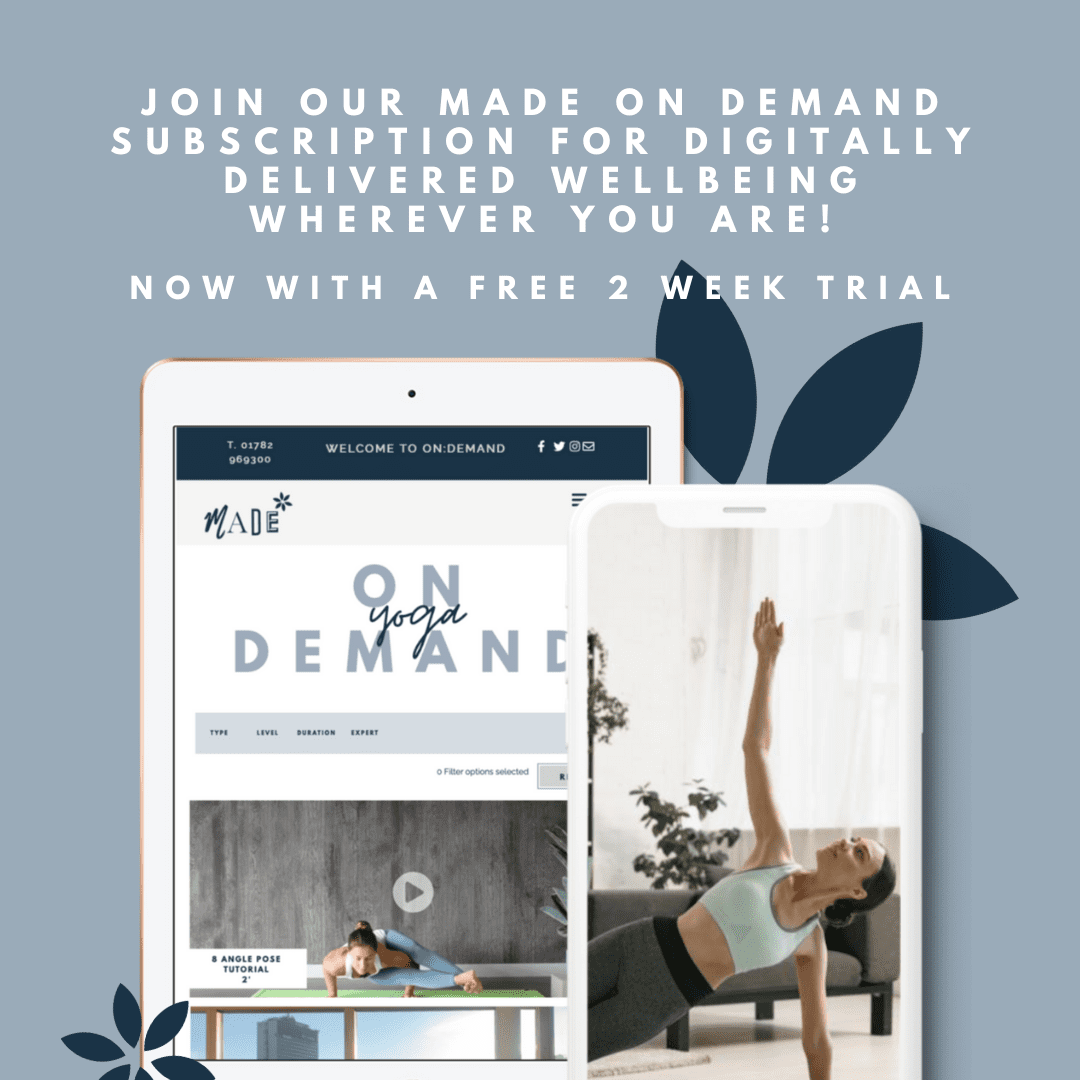The image features a square with a medium gray background. At the top, there is a prominent white text that reads, "Join our made-on-demand subscription for digitally delivered well-being wherever you are! Now with a free two-week trial." Adjacent to the text on the right side, there are dark blue leaf graphics adding a touch of nature-inspired design. 

Towards the bottom of the image, a smaller dark blue leaf print mirrors the design at the top for visual balance.

Central to the image, there is a graphic of a tablet resembling an iPad, displaying a welcome banner with the text, "Welcome to On Demand." Below the banner, the main screen focuses on a white background with a floral motif, showcasing the service "On Demand Yoga." A video player is also displayed, indicating multimedia content availability.

Next to the tablet, on the right side, there is an illustration of a white smartphone. The smartphone screen displays an image of a woman performing a yoga pose in a well-decorated living room. The background details include lush green plants, modern furniture, and a window adorned with sheer curtains cascading from top to bottom, although partially cut off at the bottom.